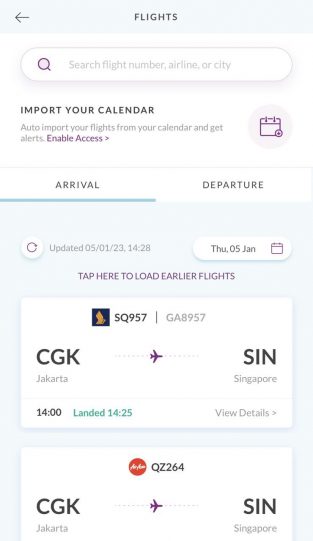The screen capture displays a user interface for a flight tracking application. At the top, there is a pale blue header featuring a gray back arrow on the left and the text "Flights" in gray. Below the header, a search box is present with a magnifying glass icon and placeholder text that reads "Search flight number, airline, or city."

Further down, there is an option labeled "Import your calendar" with the subtitle "Auto import your flights from your calendar and get alerts." An "Enable access" button in plum color, complemented with a plum calendar icon, is positioned beside this section. This is followed by a thin gray line dividing the sections.

The next section is titled "Arrival and Departure" in black, with a blue underline indicating the "Arrival" tab is active. Information at the bottom of this section states, "Last updated May 1st, 2023, 14:28," accompanied by a plum-colored refresh button. Another header reads "Thursday, 5th of Jan" with a plum calendar icon next to it, followed by a prompt in plum color that states "Tap here to load earlier flights."

The main content area starts with a navy blue box featuring a gold icon and the flight number "SQ957" in white, followed by "GA8957" in gray. Below this, details of the flight route "CGK Jakarta to SIN Singapore" are displayed with a purple airplane icon, accompanied by the scheduled time "14:00" and the status "Landed 14:25" in green.

Further down, another box is outlined with a red circle and white font displaying the flight number "QZ264." This flight also travels from "CGK Jakarta to SIN Singapore" and includes a purple airplane icon.

The image is clear and easy to read, with only a slight hint of blurriness.